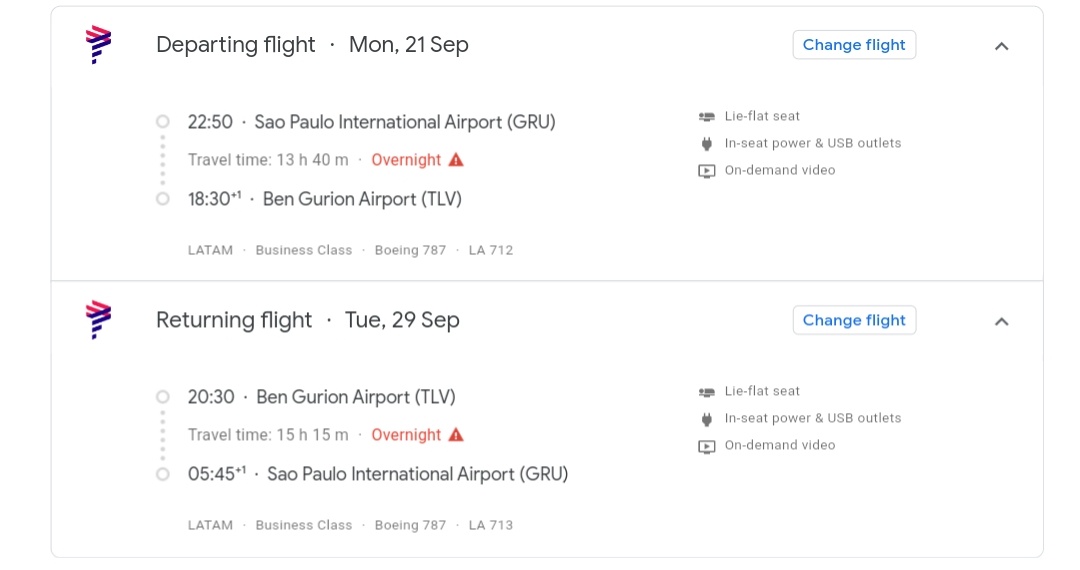**Caption:**

A detailed list of flights is displayed. 

**Departure:**  
- **Date:** Monday, 21st of September  
- **Time:** 22:50 (Military Time)  
- **From:** Sao Paolo International Airport (GRU)  
- **To:** Ben Gurion Airport in Tel Aviv (TLV)  
- **Duration:** 13 hours and 40 minutes (overnight)  
- **Class:** Business Class  
- **Aircraft:** Boeing 767  
- **Flight Number:** LA-712  
- **Amenities:** Lie-flat seat, in-seat power, USB outlets, on-demand video

**Symbol:** A red and blue swirl resembling a tornado

**Return Flight:**
- **Date:** Tuesday, 29th of September  
- **From:** Ben Gurion Airport in Tel Aviv (TLV)  
- **Travel Time:** 15 hours and 15 minutes (overnight)  
- **Arrival Time:** 5:45 (local time) at Sao Paolo International Airport  
- **Class:** Business Class  
- **Aircraft:** Boeing 767  
- **Amenities:** Lie-flat seat, in-seat power, USB outlets, on-demand video